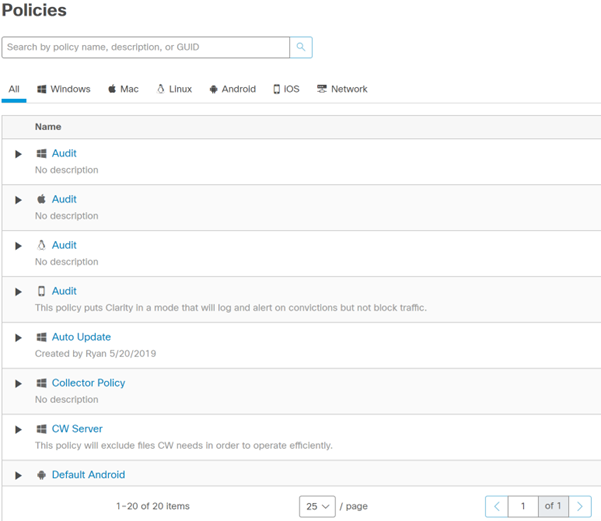**Comprehensive Policy Overview Table**

This detailed policy overview table includes multiple sections and columns for various platforms and configurations:

- **Supported Platforms:**
  - Windows (symbol: Windows)
  - Mac
  - Linux
  - Android (symbol: Android)
  - iOS
  - Network

- **Table Sections:**
  - **Main Section:**
    - **Headers:** Name, Audit, Description
    - No descriptions provided in this section.
    - **Apple Section:**
      - Headers: Apple, Audit, Description
      - No descriptions provided here either.
    - **Additional Rows:**
      - Headers: Row, Audit, Description, Audit

- **Smartphone Symbol Section:**
  - A specific row depicting a smartphone symbol with a policy that places clarity in a mode that will log and learn from convictions but will not block the traffic.

- **Auto Update Section:**
  - Windows symbol present indicating an automatic update feature.

- **Creation Details:**
  - Created by: Ryan
  - Creation Date: May 20, 2019
  - Policy Type: Collective Policy
  - Description: Not provided

- **CW Server Section:**
  - Policy Explanation: This policy will exclude files required by CW to operate efficiently.

- **Pagination and Navigation:**
  - Items Displayed: 1 to 20 of 20 items
  - Items per Page: 25
  - Page: 1 of 1
  - Navigation Arrows: Left arrow and right arrow

The above table consolidates various policies, supported platforms, and specific configuration details that are essential for system and network administration, offering a thorough view of the collective policy created on May 20, 2019, by Ryan.